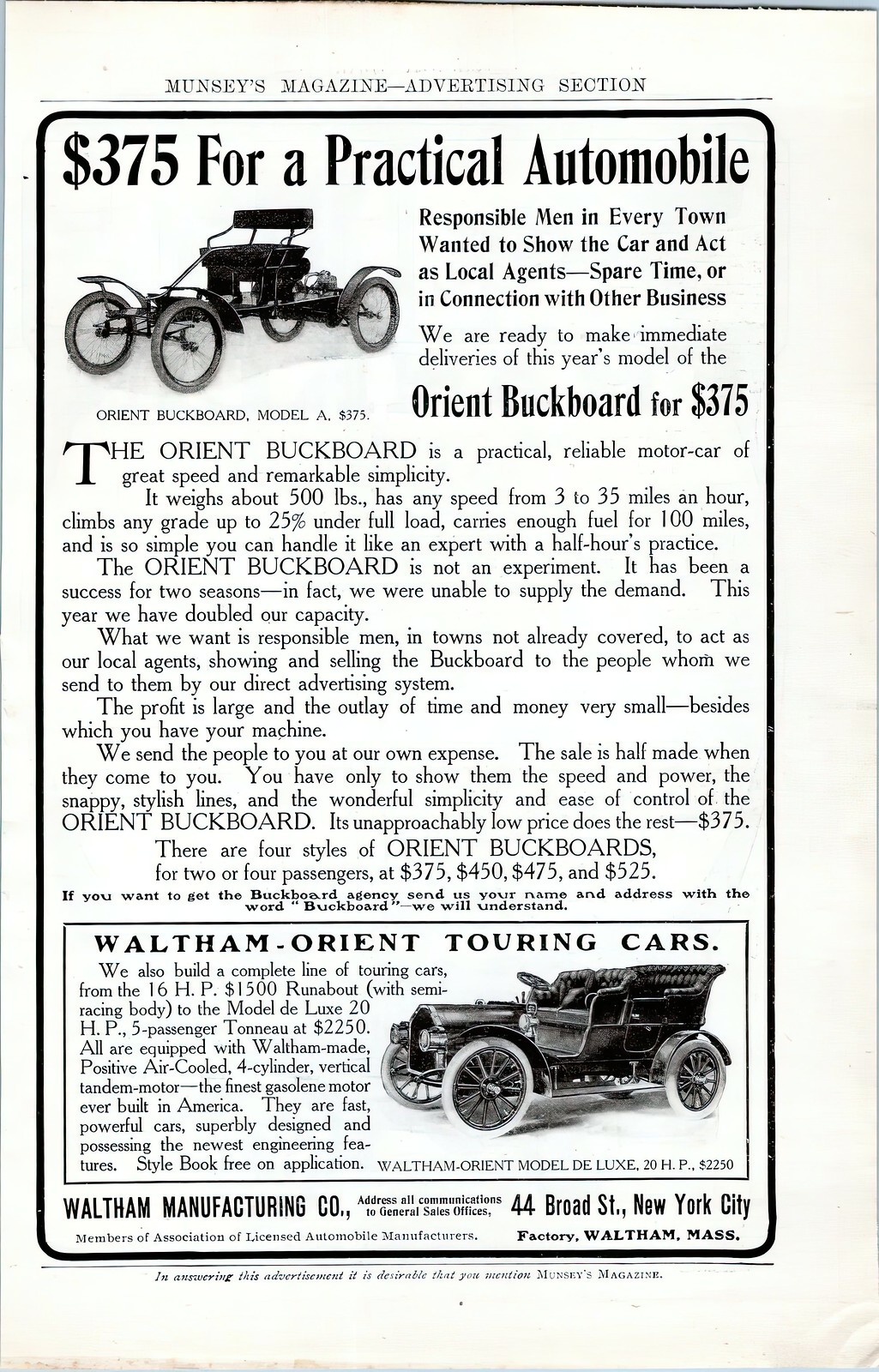This black and white photograph captures an old advertisement, likely from the 1920s, featured in Munsey's Magazine advertising section. It promotes the Orient Buckboard, an early automobile of notable simplicity and reliability. The headline at the top reads, "$375 for a practical automobile," emphasizing its affordability. The advertisement seeks responsible men in every town to act as local agents, showcasing and selling the vehicle, with opportunities for significant profit and minimal time investment. 

The Orient Buckboard is described as a practical, reliable motor car with a weight of about 500 lbs. It boasts speeds ranging from 3 to 35 mph, the ability to climb grades up to 25% under a full load, and has a fuel capacity sufficient for 100 miles. A highlight of the advertisement is the claim that the car is so user-friendly that one can become proficient with just half an hour's practice. "The Orient Buckboard is not an experiment," the text assures, underlining its success over two seasons, with the company having doubled its production capacity to meet the high demand.

The page layout includes multiple photographs of the cars. The top left features an image of a basic Orient Buckboard model, which appears minimalistic with a single row of seats and no enclosed body. Another image on the bottom right showcases a more luxurious variant with a fuller body and two rows of seats. The caption under the bottom image reads, "Waltham Orient Touring Cars," with details pointing to the Waltham Manufacturing Co. located at 44 Broad Street, New York City.

Overall, the illustration and detailed descriptions effectively highlight the affordability, practicality, and unique features of the Orient Buckboard, aimed at attracting local agents and customers to this early marvel of automotive engineering.